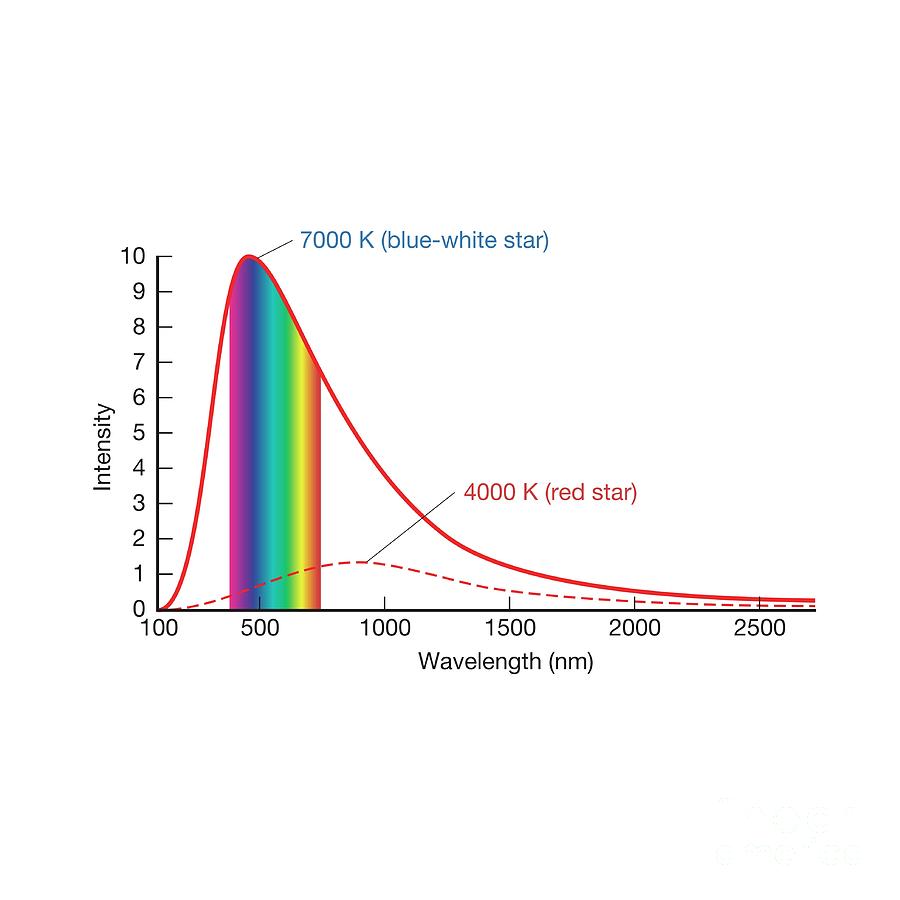The image depicts a detailed graph with the y-axis representing intensity, ranging from 0 to 10 units, and the x-axis depicting wavelength in nanometers, spanning from 100 to 2,500 nm. The graph exhibits two key plots: a solid red line representing a 7,000 Kelvin blue-white star, which peaks sharply near the 500 nm mark before tapering off towards longer wavelengths, and a dotted line denoting a 4,000 Kelvin red star, which rises more gently, peaks around 1,000 nm, and equally tapers off. The spectrum includes a visible light segment, displaying rainbow colors from purple through blue, green, yellow, and red. There's an indication of the wavelengths by color gradations between approximately 400 to 700 nm. The graph’s labels confirm that it's measuring light intensity versus wavelength, capturing the intensity variations across different temperatures of stellar objects.